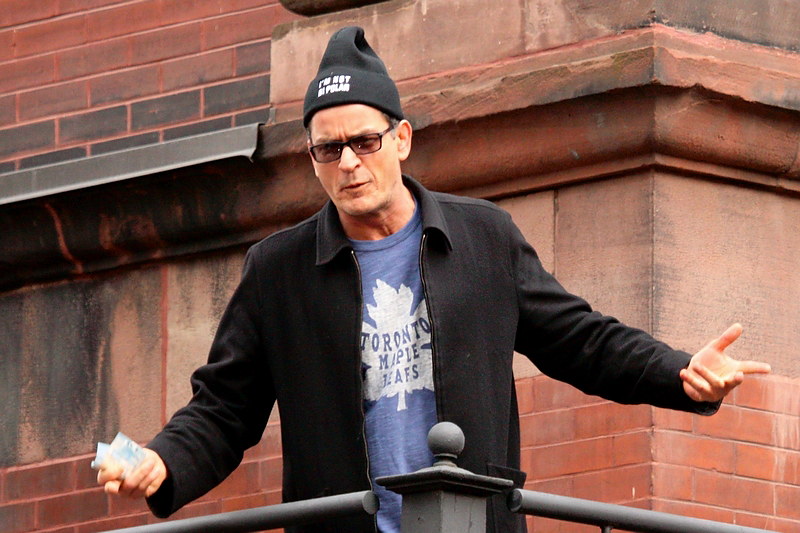In this outdoor photograph, actor Charlie Sheen stands on a balcony with his arms extended in an expressive shrug, as if questioning or addressing someone. He is dressed in a black jacket over a blue t-shirt emblazoned with a white maple leaf and the text "Toronto Maple Leafs." On his head is a black beanie with white lettering that appears to read "I'm not bipolar." Sheen is also wearing square, black-rimmed glasses with a purplish-red tint. In his right hand, which is positioned on the left side of the image, he holds a couple of cards or similar objects. Behind him, a railing borders a red brick building marred by blackened, tarnished spots.